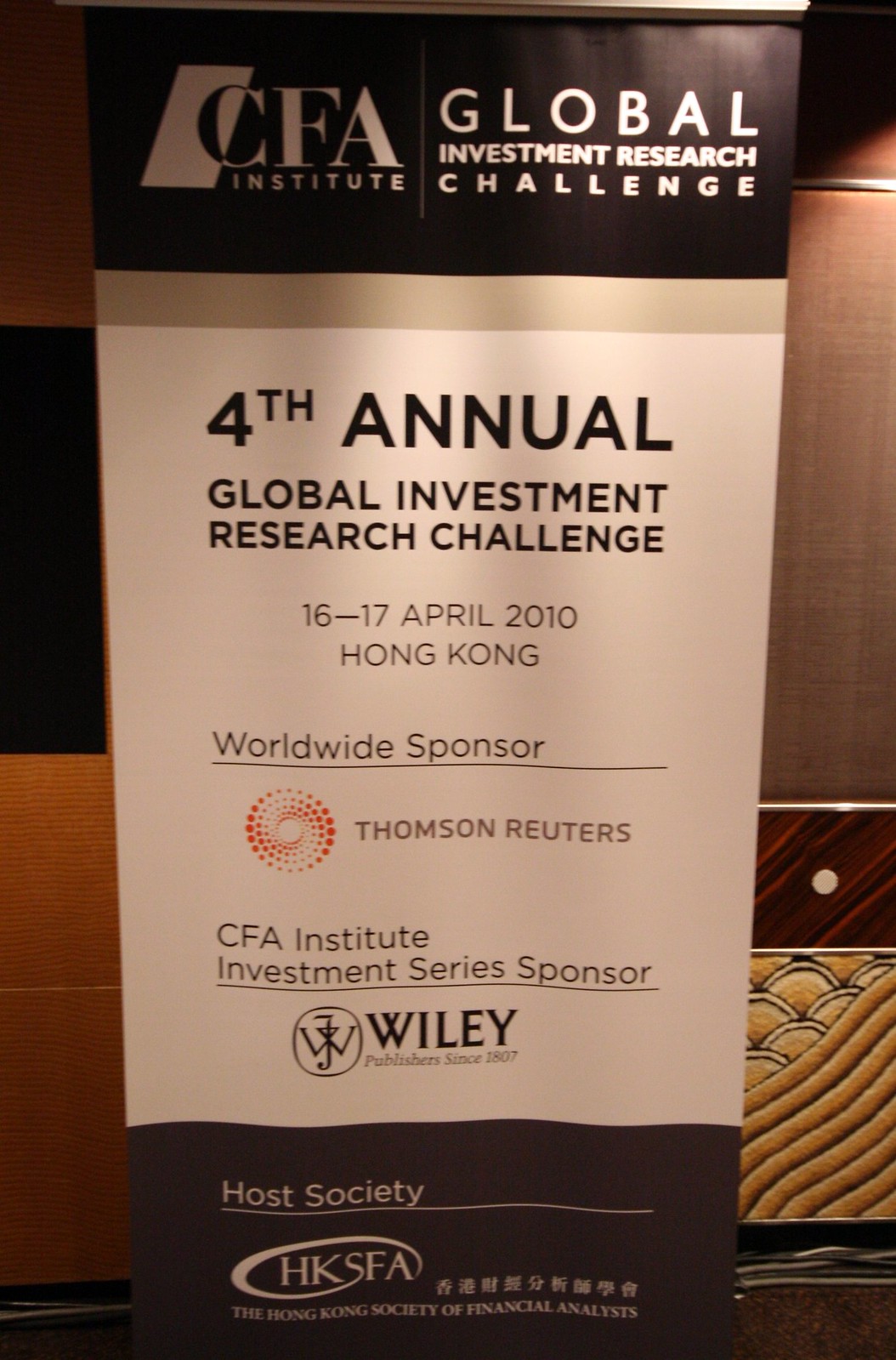The image depicts an indoor photo of a long rectangular banner set against a brown wall, with a mix of dark and light brown semi-circle and yellow light patterns along the bottom right of the wall. The top of the banner features a black section with the text "CFA Institute" and "Global Investment Research Challenge" in white letters, the former being part of a logo where the "CFA" is enclosed in a curved or tilted rectangle that inverts its colors from silver to black. 

Below this black section, the banner transitions to a white background displaying the text, "Fourth Annual Global Investment Research Challenge," followed by the date, "16 to 17 April 2010, Hong Kong." Below this information, it states "Worldwide Sponsor" and features the logo for Thomson Reuters—a circular arrangement of red dots of varying sizes forming a whirlpool shape. 

Underneath the Thomson Reuters section, the text reads "CFA Institute Investment Series Sponsor." It's further underlined, leading to the section below that features another sponsor, "Wiley," with its logo—a capital "W" intertwined with a "J." The bottom portion of the banner, reverting to a brown background, reads "Host Society HKSFA," accompanied by the text "the Hong Kong Society of Financial Analysts" and some Asian script. The banner is visually aligned to convey a sense of collaboration and sponsorship for the Global Investment Research Challenge event held in Hong Kong.